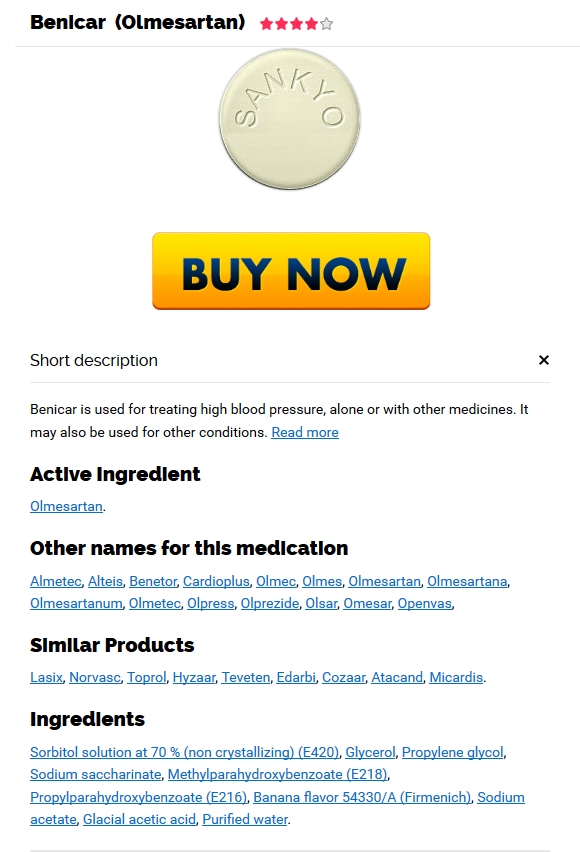The image is a vertical rectangular frame showcasing an item listing for the medication Benicar. In the top left corner, on a white background, the name "Benicar" is displayed in black with its active ingredient "Olmesartan" spelled out in parentheses (O-L-M-E-S-A-R-T-A-N). To the right of the medication name is a star rating of 4 out of 5 stars. 

Centrally placed beneath the name and rating, there is an image of the pill, which is almost ecru in color and has "Sankyo" (S-A-N-K-Y-O) imprinted on it. Below the pill image, a prominent "Buy Now" button is visible. Further down, aligned to the left, there is a section labeled "Short Description," which states: "Benicar is used for treating high blood pressure, alone or with other medicines. It may also be used for other conditions." 

Following this description is a "Read More" link, allowing users to get further information. Next, there is an "Active Ingredient" link leading to details about Olmesartan. Additionally, a section titled "Other Names for this medication" provides links to several equivalent medications. Towards the bottom, a "Similar Products" section offers links to products related to Benicar, and finally, there is an "Ingredients" link that provides detailed ingredient information.